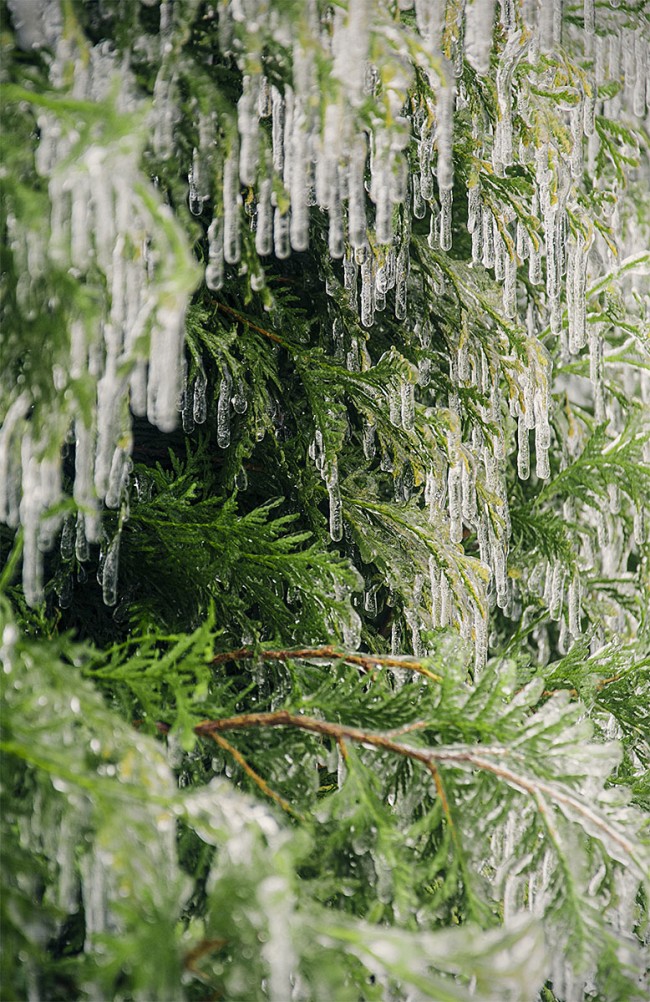This is a color photograph of a close-up view of an evergreen tree, likely a fir or pine, adorned in a wintry setting. The tree fills the entire vertical, rectangular frame of the image, with green needles and brown woody branches prominently displayed. Icicles, resembling stalactites, are hanging from the branches, formed by the slow melting and freezing of water. Most branches, especially those in the forefront, are heavily laden with clear, white, and gray icicles, creating a glistening, icy spectacle. While some branches towards the center remain exposed, the majority are enveloped in these frozen formations. The photograph showcases this frosty scene against a contrasting black background, emphasizing the intricate details of the ice-covered tree.